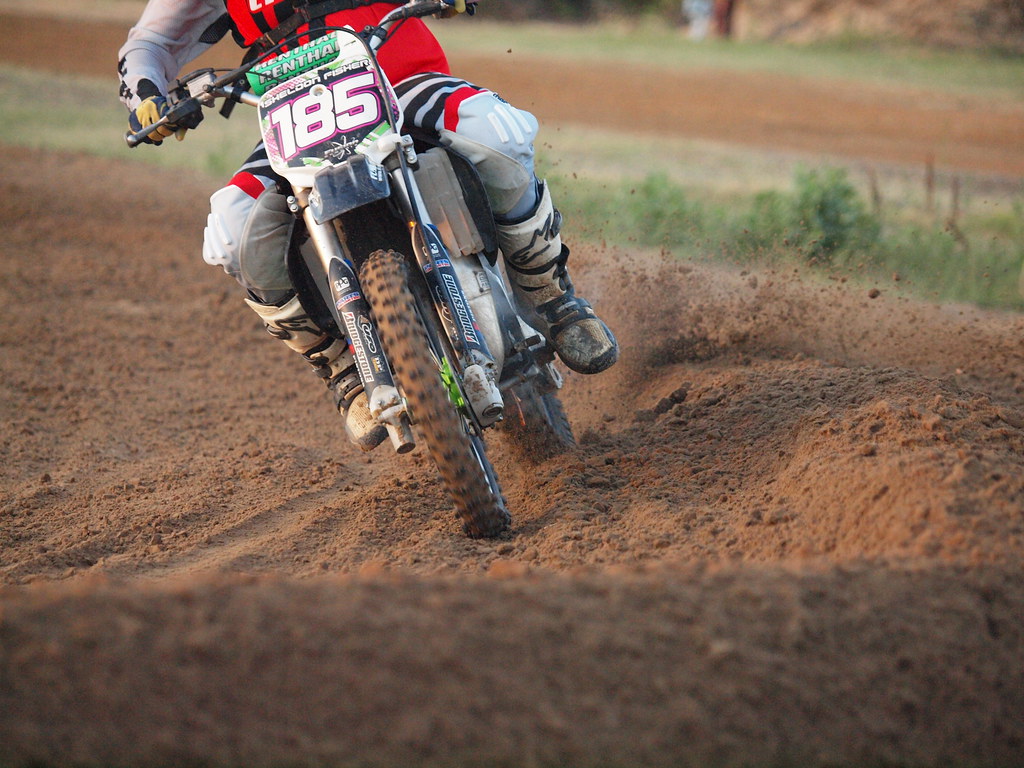A close-up action shot captures a rider named Sheldon Fisher maneuvering his dirt bike, numbered 185, around a turn on a dirt track. The rider, dressed in a distinctive red and white racing suit with black stripes, thick boots, gloves, and arm padding, is the central focus of the image. Soil is seen being flung from the back wheel, emphasizing the speed and intensity of the maneuver. The background, although blurred, hints at greenery and fields beyond the dirt path, with afternoon sunlight casting subtle highlights. The bike and rider are facing towards the camera, illustrating the precision and skill involved in the sport. This image likely originates from a formal racing event, given the detailed visible gear and numbered bike.